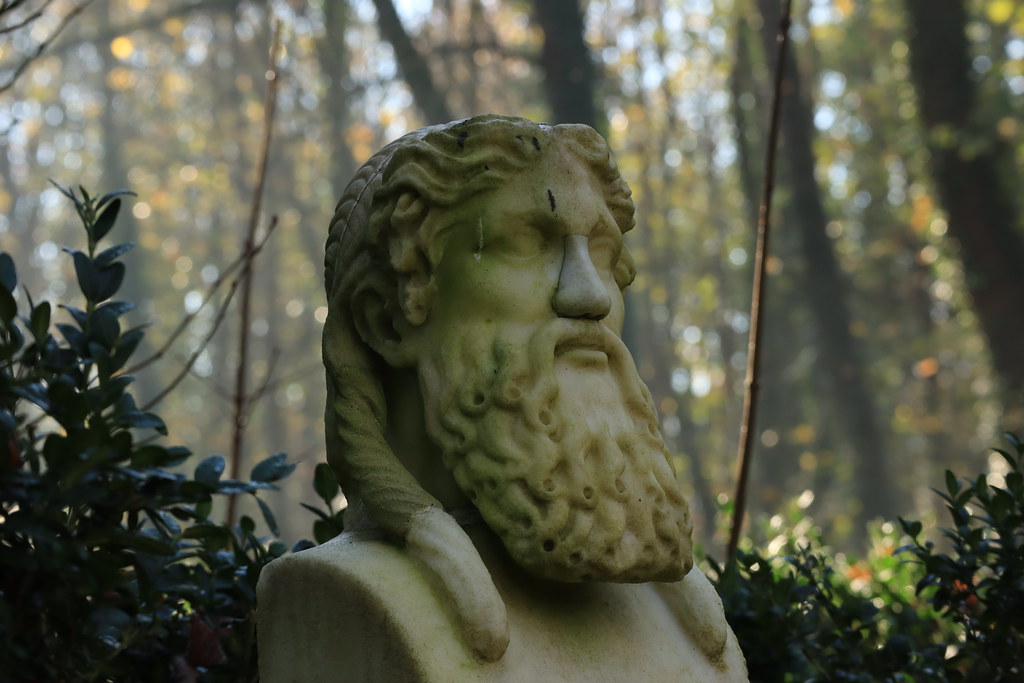The photograph depicts an ancient Greek-style bust statue of an older man with a detailed marble or plaster finish. The statue features intricately carved wavy hair and two prominent locks of longer hair cascading down to the chest area over each shoulder. He has a distinctive tubular-looking beard, roughly 10-12 centimeters in length. The stone of the statue is notably worn, showing signs of age with a greenish tint, likely due to mold or algae. The setting is outdoors in a wooded area, with low-lying bushes of deep green leaves surrounding the bust. Behind the bushes, the background becomes more blurred, revealing slender tree trunks and patches of bright blue sky peeking through the foliage. The photograph is focused on the statue, emphasizing its detailed craftsmanship and the passage of time visible in its weathered appearance.